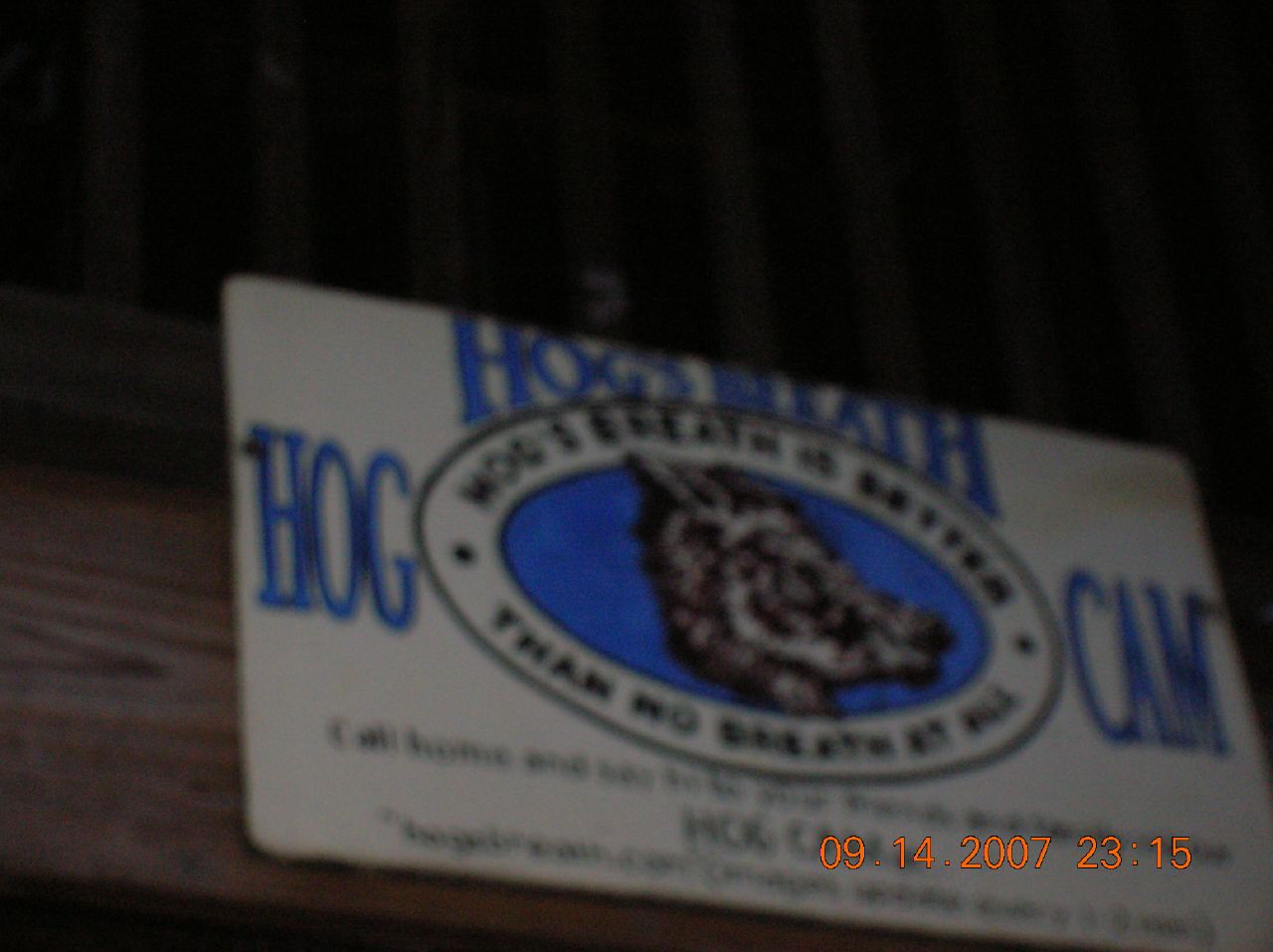The image is a blurry digital photo of a sign or fake license plate taken on September 14th, 2007 at 11:15 PM, as indicated by the orange date and time markers in the bottom right corner. The sign appears to be mounted against a wooden post or board background. At the top of the sign, though slightly unreadable, it likely reads "Hog's Breath is better than no breath at all." In the center is a horizontal oval bordered in black, containing another smaller black-bordered blue oval that features a black and white sketch of a hog's face. To the left of the oval, in big blue letters, it says "HOG," and to the right, it says "CAM," together forming "HOG CAM."